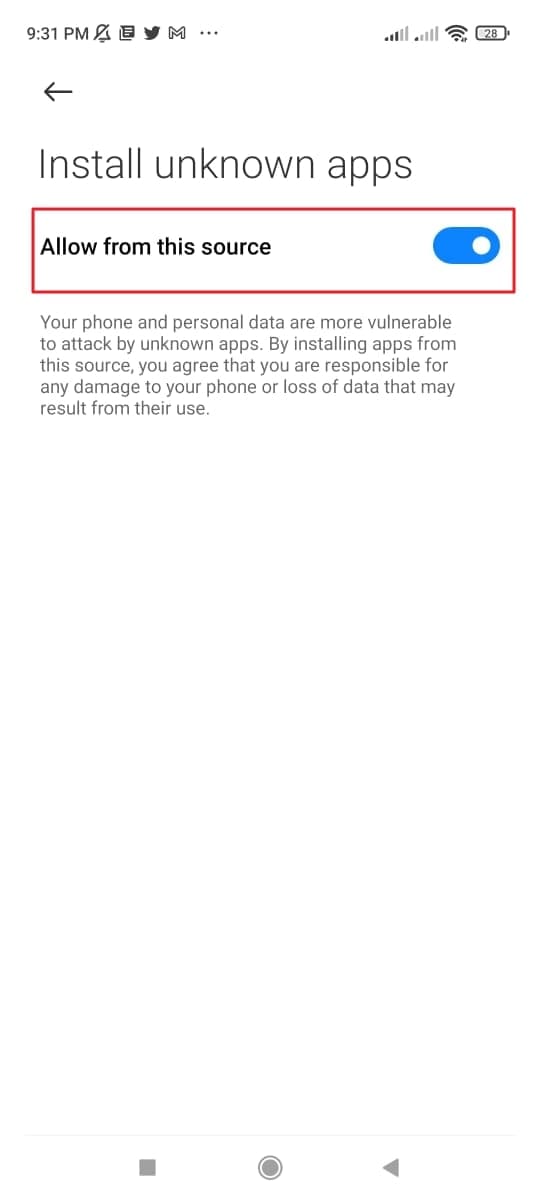Screenshot of a smartphone screen taken at 9:31 PM. At the top left, the status bar shows the time, a bell icon with a line through it indicating no notifications, and several social media icons including the Twitter bird and an 'M' in parentheses, followed by three vertical dots. On the right side of the status bar, there are two sets of signal bars; the first set has three out of five bars filled, and the second set has one out of five bars filled. The Wi-Fi icon indicates connectivity, and the battery icon shows it at 25% charge.

Below the status bar, a back arrow points to the left, below which is the heading "Install Unknown Apps" displayed prominently. A white bar outlined in red underneath the heading contains the text "Allow from this source" in bold, with a blue toggle switch on the right side that is currently switched on. A warning message follows: "Your phone and personal data are more vulnerable to attack by unknown apps. By installing apps from this source, you agree that you are responsible for any damage to your phone or loss of data that may result from their use."

At the bottom of the screen, there are three icons: a gray rectangular back button on the left, a gray circular home button in the center, and a gray left-facing caret symbol on the right.